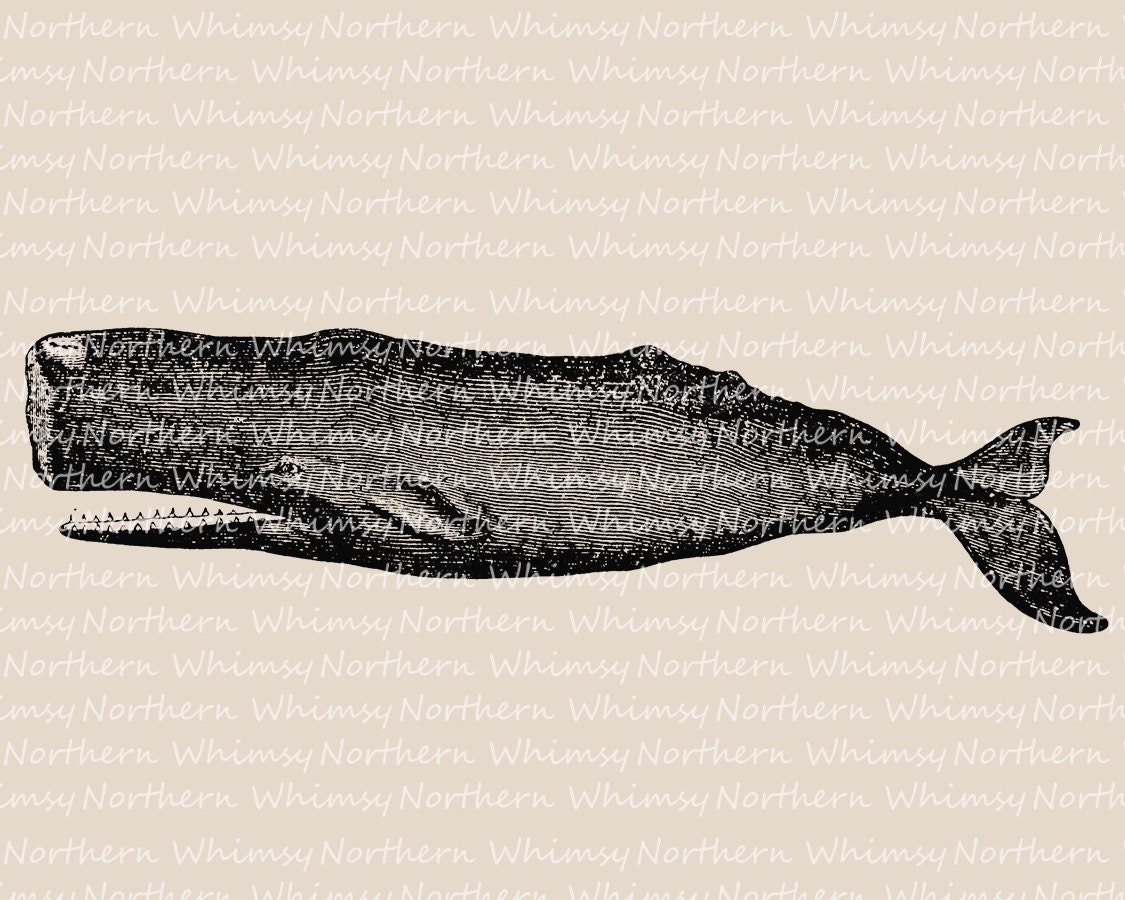A light tan or pale lavender background frames a single, large whale positioned centrally in the image. The entire picture is overlaid with repetitive text in white that reads "Whimzee Northern," creating an intricate pattern that covers both the whale and the background. The text, forming continuous lines, fills up the entire frame from top to bottom, making it somewhat challenging to read due to the background color.

The whale itself appears to be a pencil drawing with bold, black charcoal lines, giving it a detailed and textured look. It is depicted in a side view, facing to the left, with its square snout, single visible eye, and mouth wide open, revealing an array of sharp, lower teeth. The whale's body stretches from the tail, which has a short, double fin, all the way to the forefront snout, and horizontal stripes run across its body. Despite its menacing teeth and large size, there is a whimsy to the drawing that aligns with the textual overlay. The creature illustrated is likely extinct, recognizable for its unique features and sketched appearance, edged boldly to stand out amidst the repetitive text.